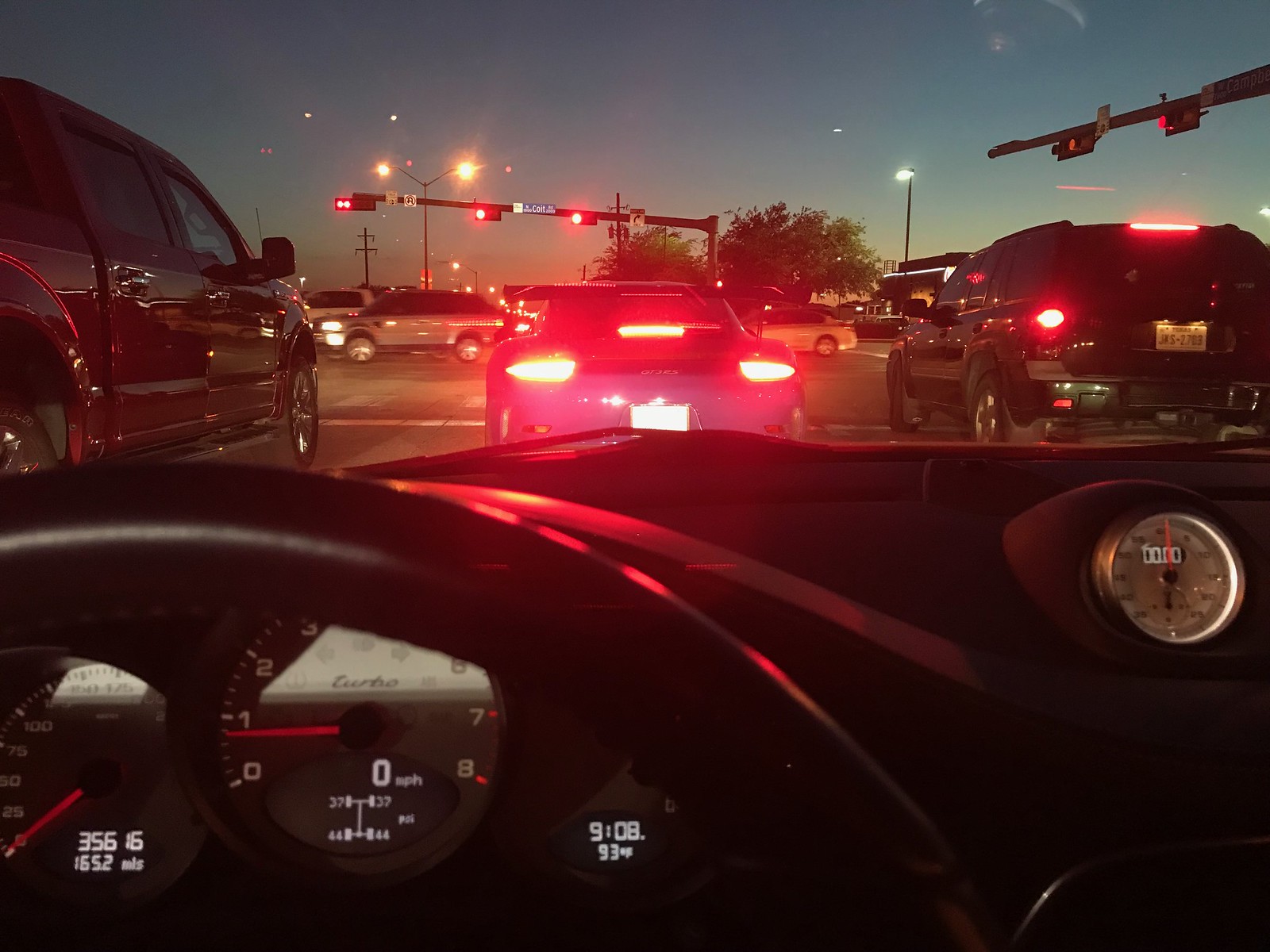The image depicts the interior of a vehicle, featuring a prominent black leather steering wheel at the forefront. The dashboard is equipped with several indicators, including a central speedometer with a red needle pointed at the "1" mark. To the right of the speedometer, a digital display reads "9.08," while another indicator shows an outside temperature of 93 degrees Fahrenheit. Additionally, there is a clock face on the dashboard's center, displaying "0000" with a red arrow pointing upwards and white numerals.

In the background, the scene outside the vehicle is visible through the windshield. On the left, there is a red truck, and in the middle, a blue car with red taillights. On the right, a black truck can be seen. The setting includes traffic lights in the top right corner of the image, displaying red lights at the far end. Above, the sky is clear and blue, adding to the scene's atmosphere.